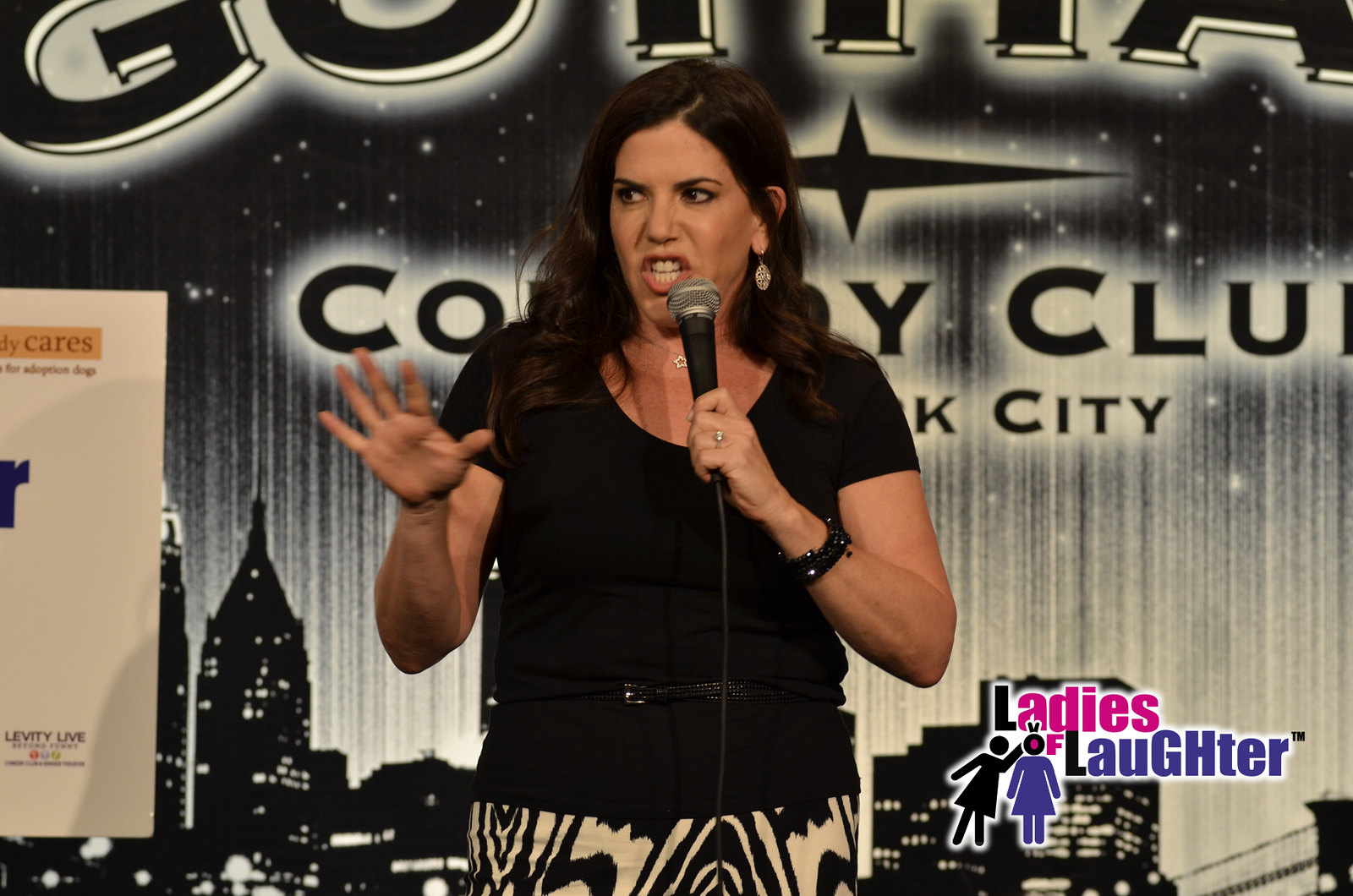The image captures a dynamic moment of a female comedian performing on stage, likely at Gotham Comedy Club in New York City. Central to the composition, the woman is animatedly speaking into a microphone, emphasizing her expressive delivery. She has long dark hair, appears to be in her 30s, and is wearing a black short-sleeved blouse paired with black and white striped pants. Her attire is accessorized with a black bracelet, a diamond ring, star-studded necklace, and earrings. The background showcases an artistic depiction of a city skyline with white rays extending upwards, accentuating the venue's branding, including partially visible text indicating "Gotham Comedy Club" and "New York City." Notably, the bottom right corner of the image features the logo and caption "Ladies of Laughter," accompanied by an icon of two female stick figures.